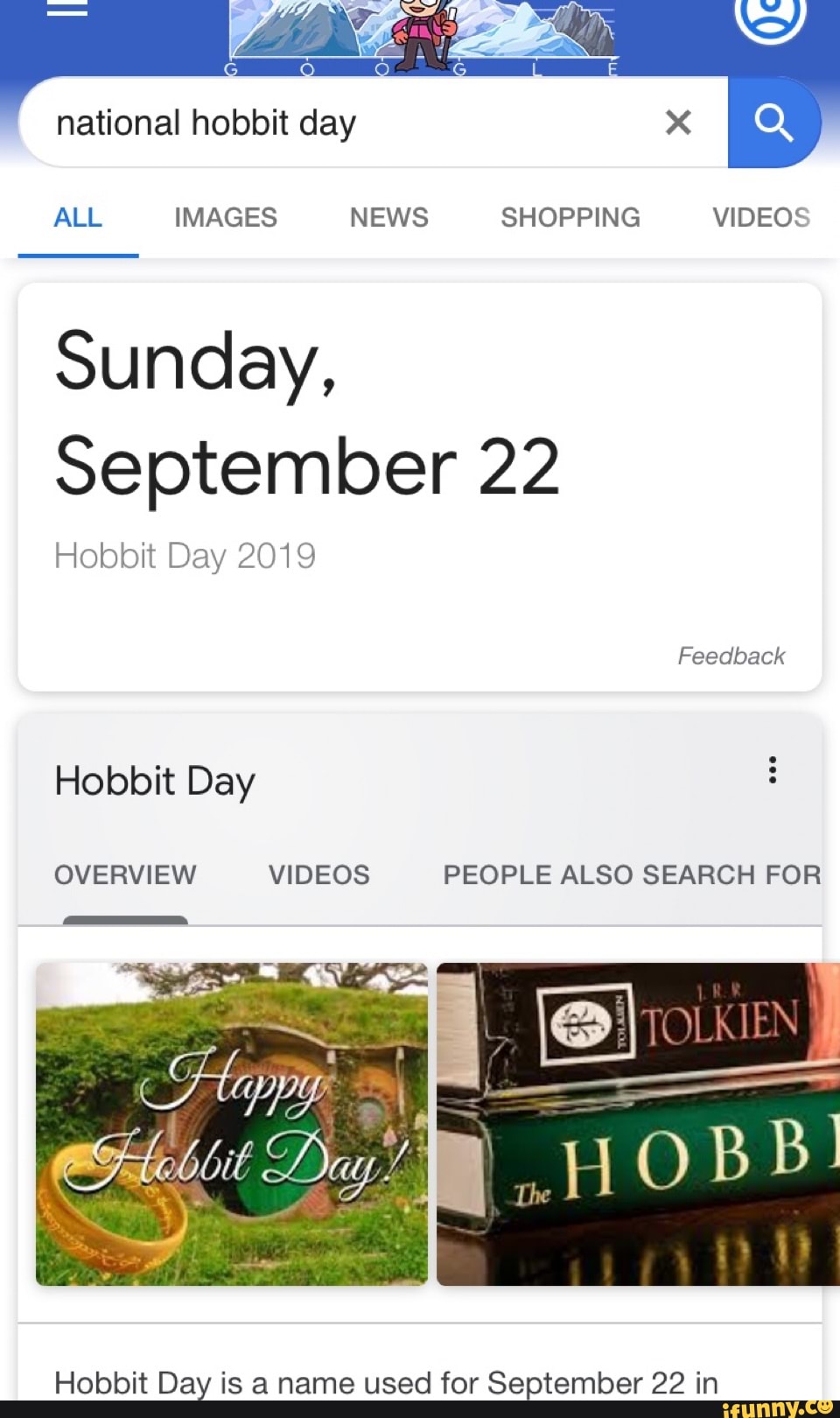A phone screen displays a Google Chrome browser where a search for "National Hobbit Day" has been conducted. The top search result indicates that Hobbit Day falls on Sunday, September 22, 2019. Below this, further search results related to Hobbit Day are visible. The first result features an image with the caption "Happy Hobbit Day," showcasing a picturesque hobbit home embedded into a grassy hillside with an overlay image of the iconic Lord of the Rings ring in front of the dwelling. To the right of this image, there are two books displayed: one titled "J. R. R. Tolkien" and the other "The Hobbit." The text explains that Hobbit Day is celebrated on September 22nd. This detailed search effectively provides information about the specific date of Hobbit Day in 2019, confirming it as a single day event rather than every Sunday in September.